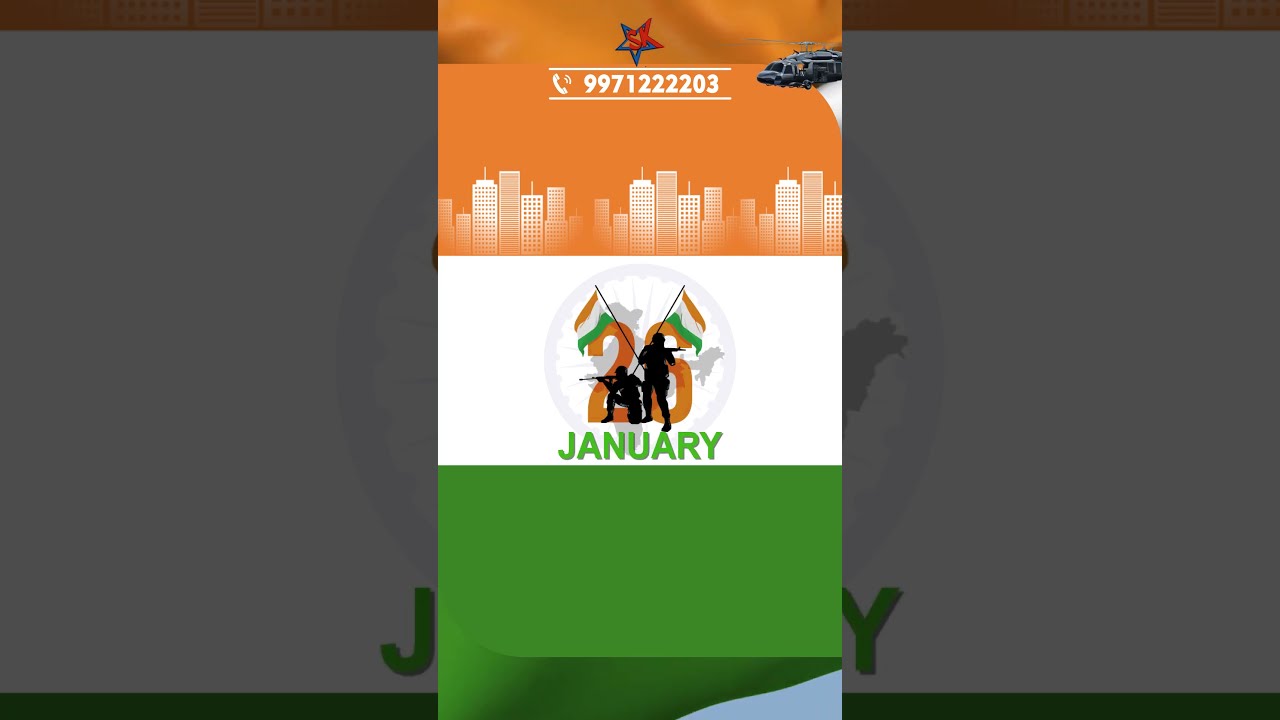The image is divided into three distinct sections featuring a tricolor scheme of orange, white, and green. The top portion of the image is orange, displaying a city landscape created in an art illustration style with white skyscrapers and buildings. Above this cityscape, there's a phone number, 997-122-2203, and a star rendered in red and blue, situated towards the middle. On the upper right side, there is an illustration of a helicopter. 

Below the orange section, the middle strip of the image is white, prominently displaying the date "26 January" in orange and green text. This middle section also features two black silhouette soldiers holding rifles – one standing, the other kneeling – with two crisscrossed flags behind them. The lower section of the image is entirely green with no additional content. The overall colorful composition and elements suggest the image might be related to commemorating a holiday or special event.